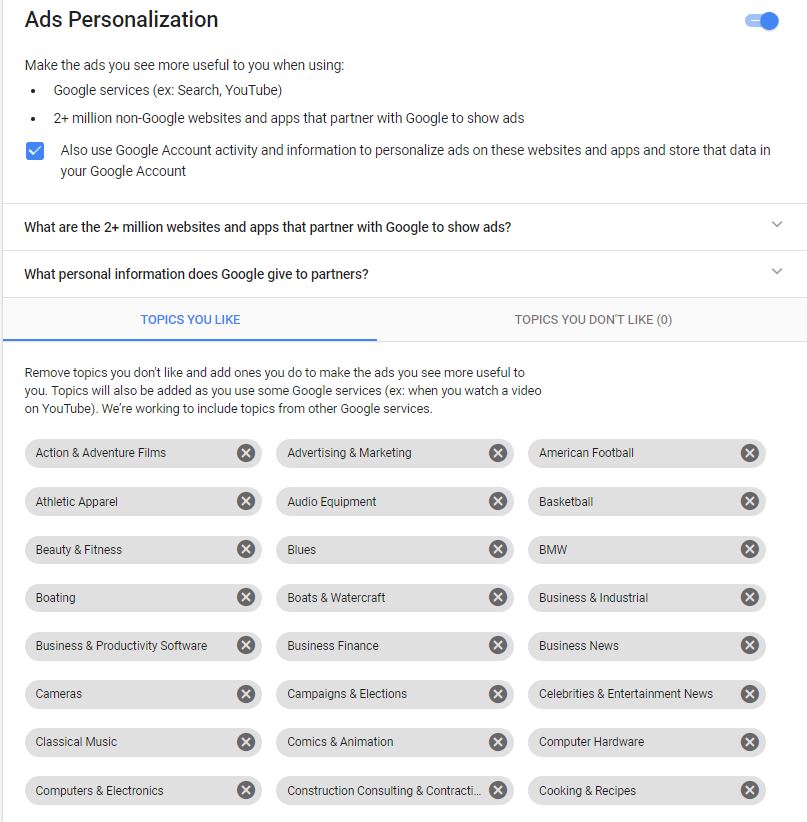**Image Caption:**

The screenshot illustrates Google's ad personalization interface, guiding users on how to optimize their ad experience across Google's services and its extensive partner network of over 2 million websites. At the top, users are informed about the benefits of personalizing ads, including making them more relevant and useful. The interface explains how Google uses connectivity information and personal data to tailor ads on various platforms such as Google Search, YouTube, and third-party sites.

A comprehensive list of interests is presented, allowing users to select topics they prefer, ensuring they see ads aligned with their preferences. Categories include a wide array of interests such as Action & Adventure Films, Athletic Apparel, Beauty & Fitness, Boating, Business & Productivity Software, Classical Music, Computer Electronics, Marketing, Audio Equipment, Boats & Watercraft, Business Finance, Comics & Animation, Construction & Contracting, American Football, Basketball, BMW, Business News, Celebrity Entertainment News, Computer Hardware, and Cooking Recipes.

Users can also deselect topics they are not interested in, further refining the personalization process. This detailed list allows for a highly customized advertising experience, aiming to make ads more relevant and engaging for the user.